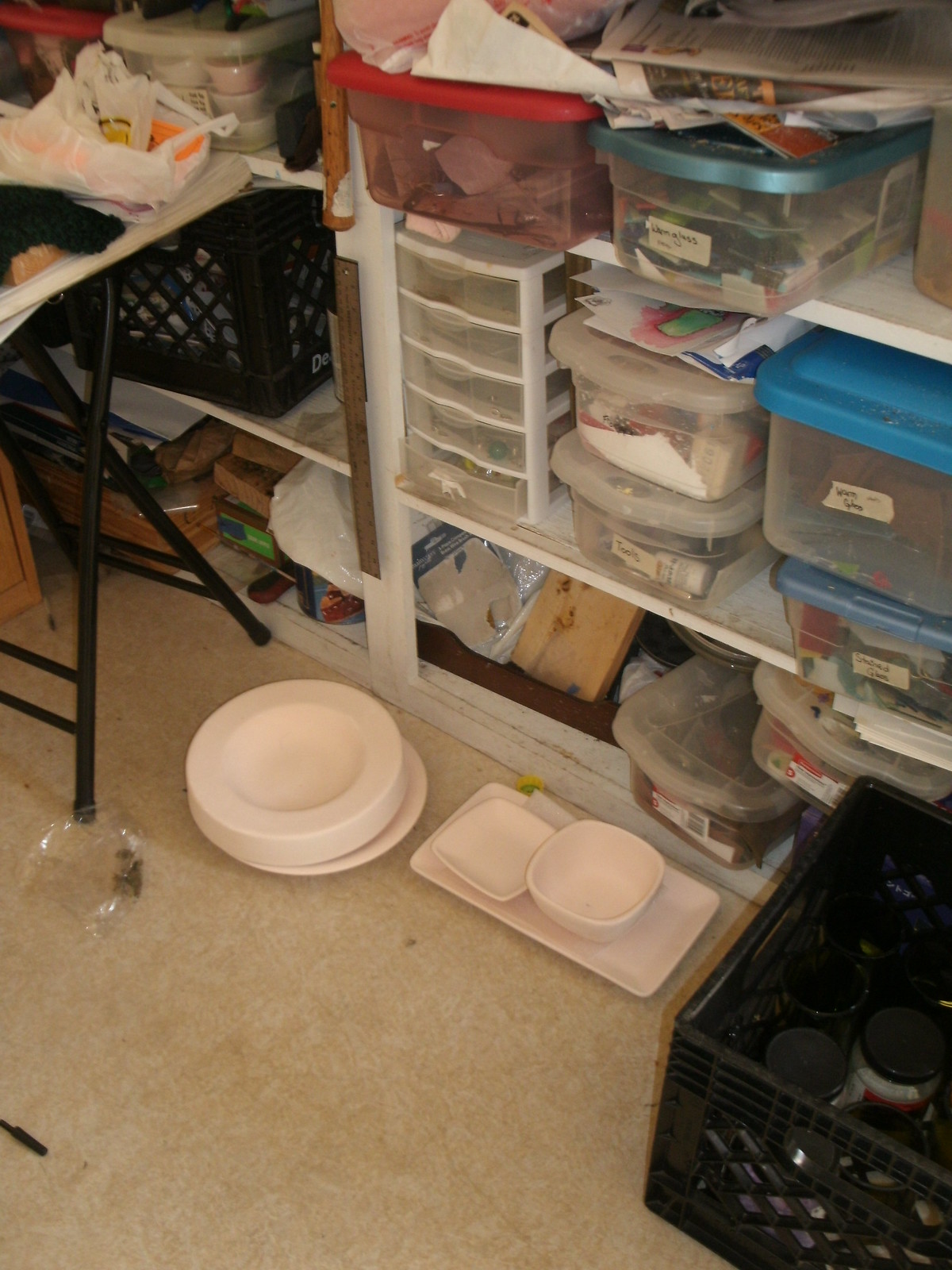This image showcases a well-organized utility room featuring white shelving units stocked with an array of plastic containers. Each container is neatly labeled with masking tape, likely containing food items such as dog and cat food. Positioned below the shelves, a white carpeted floor supports a rectangular plate holding two ceramic bowls—indicative of pet feeding stations. To the left of the feeding area, disposable paper bowls or plates are scattered on the floor. An ironing board, cluttered with various items, stands off to the far left. Resting on the shelves, a black laundry basket is visible, along with clear plastic containers adorned with blue, light blue, and red lids. Towards the bottom right, a milk carton-style plastic container filled with assorted baubles and capped with black lids can be seen. A small piece of plastic lies on the floor, completing the scene's detailed inventory.